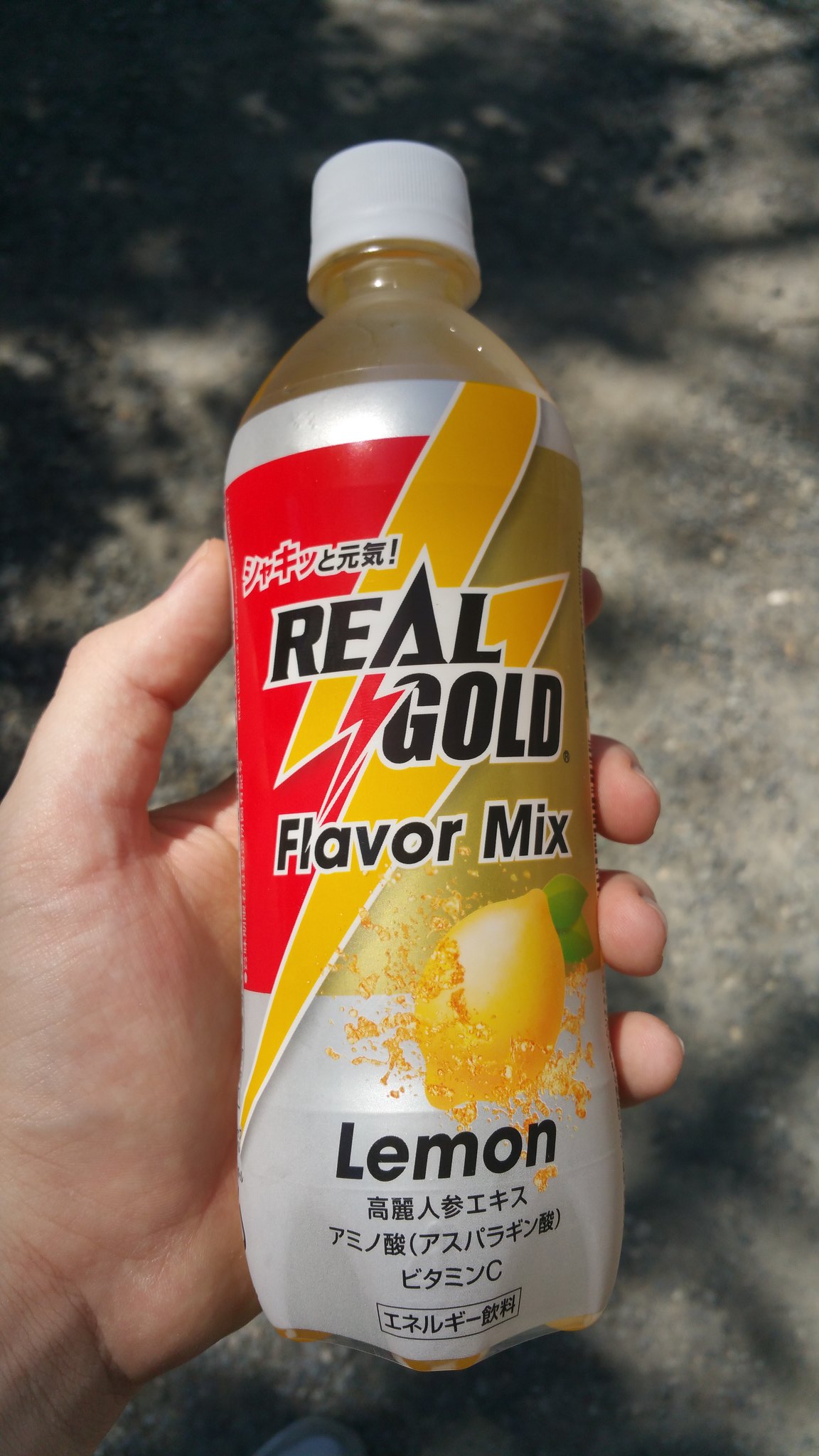This image captures a plastic beverage bottle with a white cap, prominently held in the palm of someone's hand. The main focal point is the bottle, which contains a yellowish liquid that resembles lemonade. The label on the bottle features the text "Real Gold Flavor Mix" with a bold yellow and red lightning bolt logo behind it. Below this, there's an image of a lemon with green leaves, accompanied by the word "Lemon" in black. The text at the top of the label is in Japanese, making it unreadable for those unfamiliar with the language. The photo appears to have been taken outdoors on a gray pavement, evidenced by the shadow of a tree cast on the ground in the background, despite the tree itself not being visible within the image.